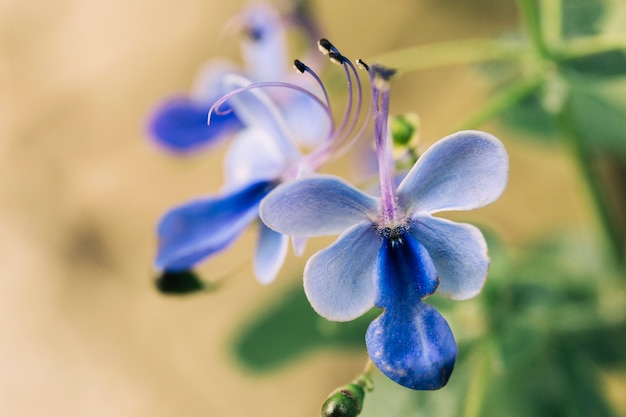The photograph showcases a vividly detailed blue orchid at its center, which is in sharp focus. This prominent bloom boasts four radiating light blue petals, with the central downward petal being a striking darker blue. The flower is adorned with two light purple stamens or pistils, extending from its core, topped with black structures. At the base of this blossom, there is a round green structure, possibly an unopened bud, signifying it may soon bloom. In the background, slightly blurred, are two more of the same blue orchids, hinting at a cluster of these beautiful flowers. The backdrop of the image carries an orangish-brown hue, with some blurred greenery and other plant types present in the right corner, contributing to the overall natural setting.